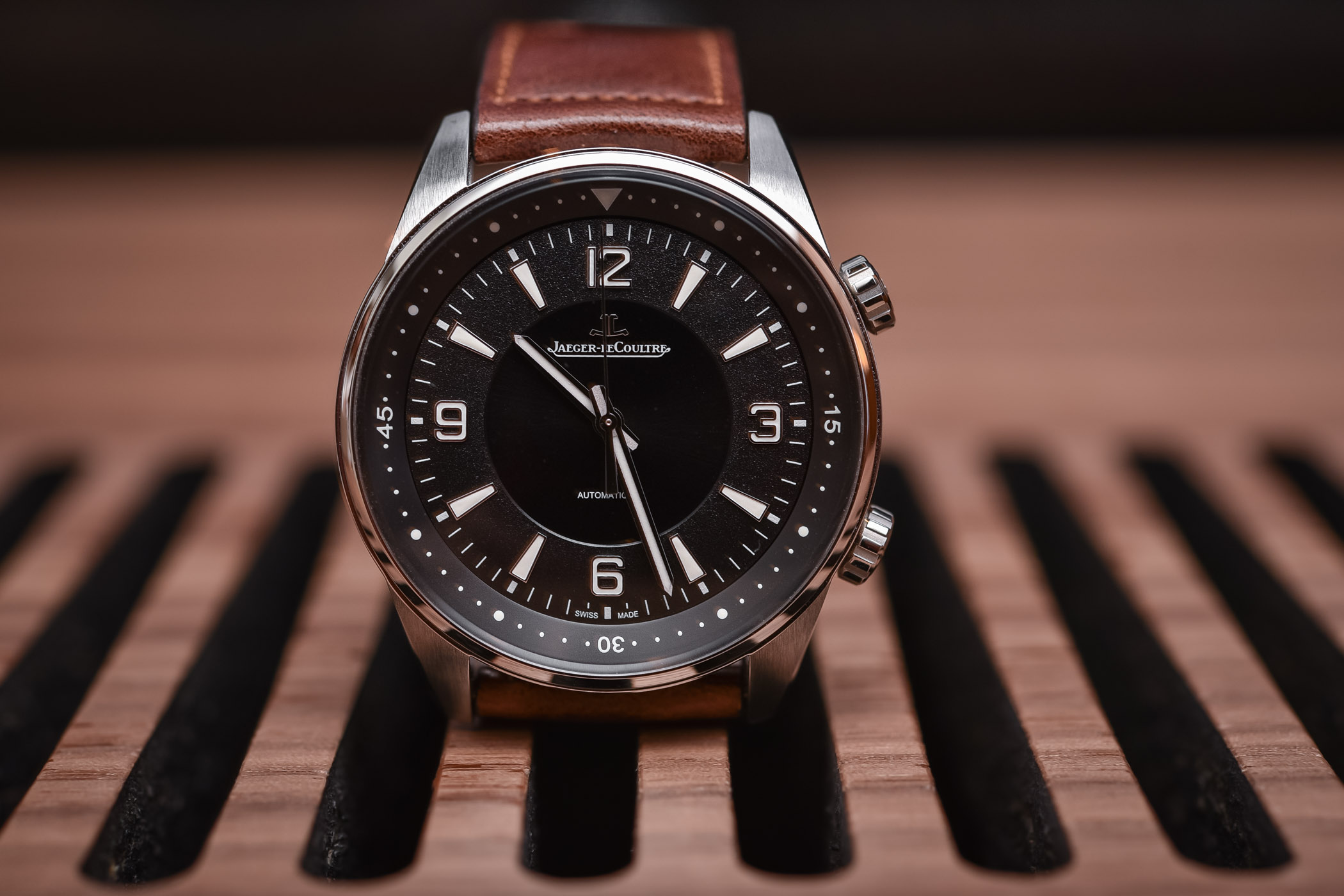This close-up, horizontal rectangular image showcases a well-crafted men's wristwatch, appearing almost as if it's part of an advertisement. The watch features a dark brown leather band and a sleek, silver casing with two buttons on the side, likely indicating stainless steel material. The analog face of the watch is predominantly black, displaying only the numbers 12, 3, 6, and 9, with minimalist dashes marking the other hours. The silver hands point to roughly 10:30. Inside the dial, subtle lettering reads "Jagger Couture," although the finer details are too small to discern clearly. The watch is elegantly positioned on a light to medium brown wooden stand, which appears to be a tray with black slats. The background of the image is artistically blurred, drawing full attention to the timepiece.